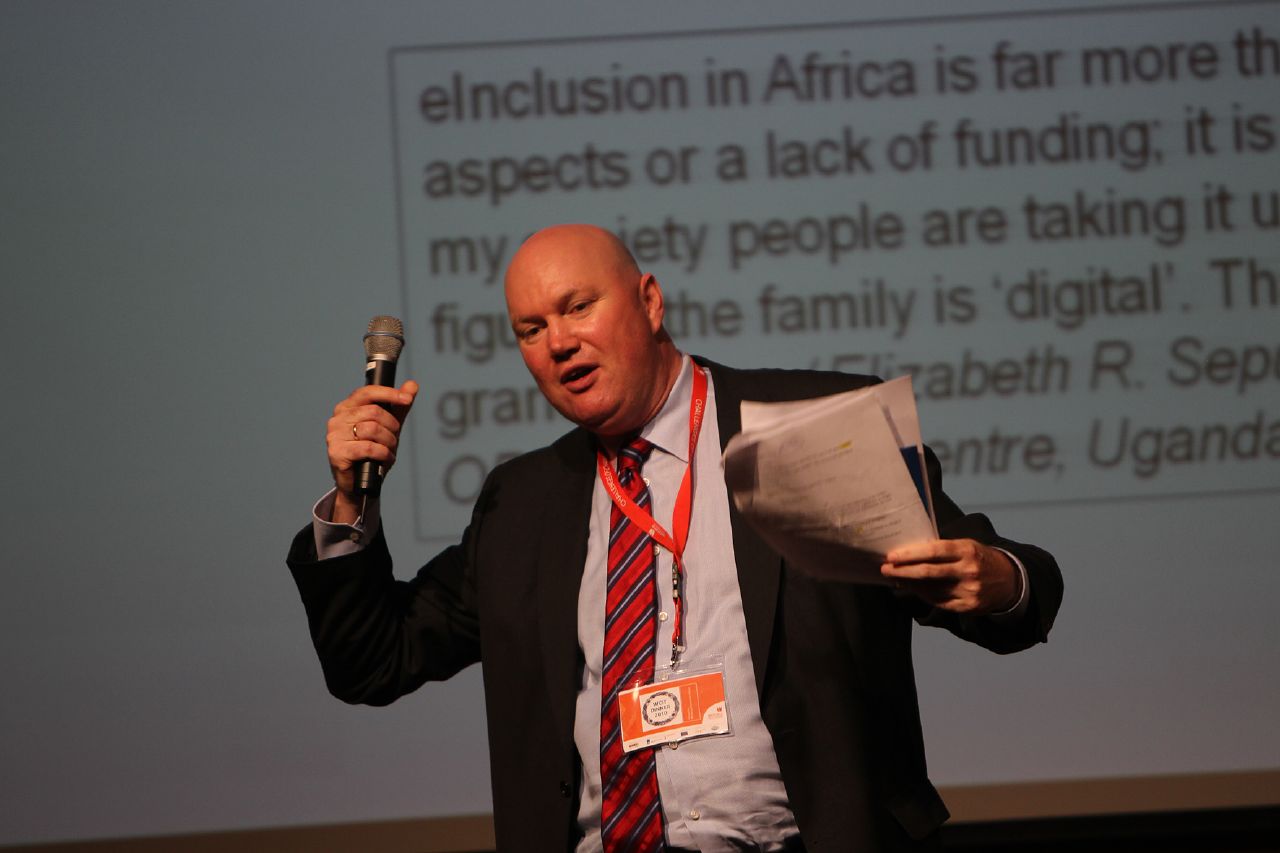In the image, a bald, slightly heavyset man is captured mid-speech. He is positioned on the right side of the frame, holding a microphone near his head with his left hand and a stack of slightly bent papers in his right hand. He appears animated, with his mouth open and head tilted slightly to the left, engaged in addressing his audience. He wears a black jacket over a white button-down shirt, adorned with a red tie featuring diagonal blue and white stripes. A lanyard with an event pass or badge hangs around his neck. Behind him, a PowerPoint slide is displayed on a whitish background, containing partially obscured text within a thin black-edged rectangle. The visible text includes phrases such as "L-E-L-N-C-L-U-S-I-O-N in Africa is far more," "aspects or lack of funding," and "the family is digital," as well as the name "Elizabeth R" and "Uganda."